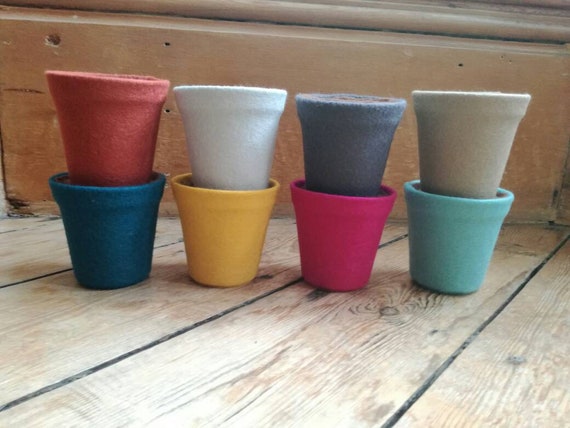The image features eight small, woven or cloth flower pots arranged in a striking manner on a wooden deck or porch with natural, spaced-out wooden boards. The pots are organized in two rows, with the bottom row consisting of four pots, and an additional four pots stacked directly on top of them. The color scheme of the pots includes teal, gray, pink, navy blue, white, yellow, a darker blue, and a peachish-orangeish-red. Specifically, the bottom left pot is teal, with a reddish-orange pot stacked on top; the next set consists of a yellow pot with a white pot on top; adjacent to that is a pink pot with a gray pot stacked above; and the final set includes a light blue pot with a beige-green pot on top. Behind the neatly arranged pots is a wooden baseboard that adds a rustic touch to the scene.